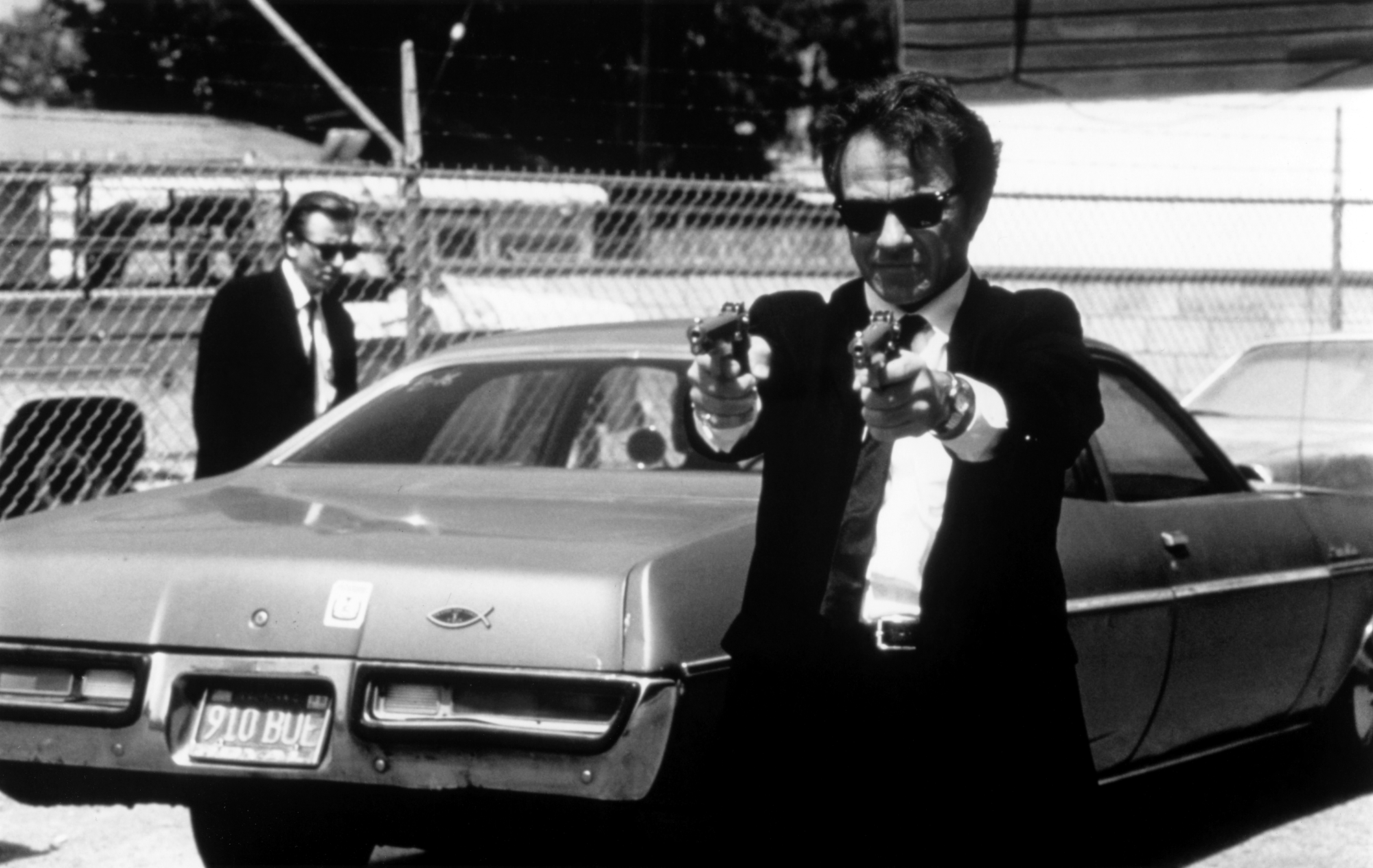The black-and-white photograph captures a dramatic scene reminiscent of a 1970s movie still. Dominating the center is a long, vintage two-door car, possibly a Monte Carlo, with a distinctive sloped design and a small Jesus fish emblem on the trunk. The vehicle bears the license plate "910 BUE." 

To the left of the car stands a man next to the driver's side door. He is poised as if about to enter, dressed in a black suit, black tie, white collared shirt, and black Wayfarer-style sunglasses. Behind the car, another man faces the camera, wearing a similar outfit. This man holds two pistols, one in each hand, aiming them menacingly towards the camera. He has short hair on the sides with a longer top and also wears dark sunglasses, giving him a composed, yet intimidating presence. The backdrop features a chain-link fence with barbed wire, and several buses are visible beyond the fence, enhancing the gritty, cinematic quality of the image.